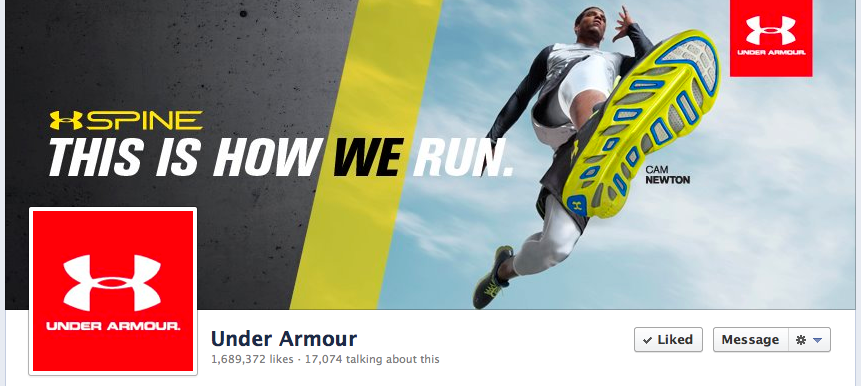The image is a promotional screenshot for an Under Armour product, specifically the "Spine" tennis shoes. The Under Armour logo appears prominently throughout the advertisement, notably in the lower left corner in red and white, accompanied by the slogan "This is how we run" in white text, except for the word "WE," which is highlighted in black. Adjacent to this text is a count of social media engagement, stating "1,689,372 likes" and "17,074 talking about this," followed by options to "Like" and "Message," and settings indicated by a gear symbol and a blue downward arrow.

Dominating the right side of the image is a dynamic photograph of an athlete captured from a low angle, giving the impression of looking upwards at him against a sky backdrop. The athlete is airborne, either jumping or running, with no ground or trees visible in the shot. He wears Under Armour "Spine" tennis shoes, which are described in detail: grey with yellow accents, a white sole interspersed with fluorescent green, blue, and grey sections, and a blue heel section featuring a yellow Under Armour logo. The shoes are laced with bright yellow shoelaces.

The athlete's attire includes white tights beneath grey shorts and a grey and white long-sleeved top. He appears to be of darker skin tone, possibly African-American, with short hair. Additional Under Armour branding is found in the upper right corner of the advertisement, featuring the logo in red and white. Notably, the athlete is identified as Cam Newton, an esteemed figure in the sports world, as indicated next to the image of the shoe.